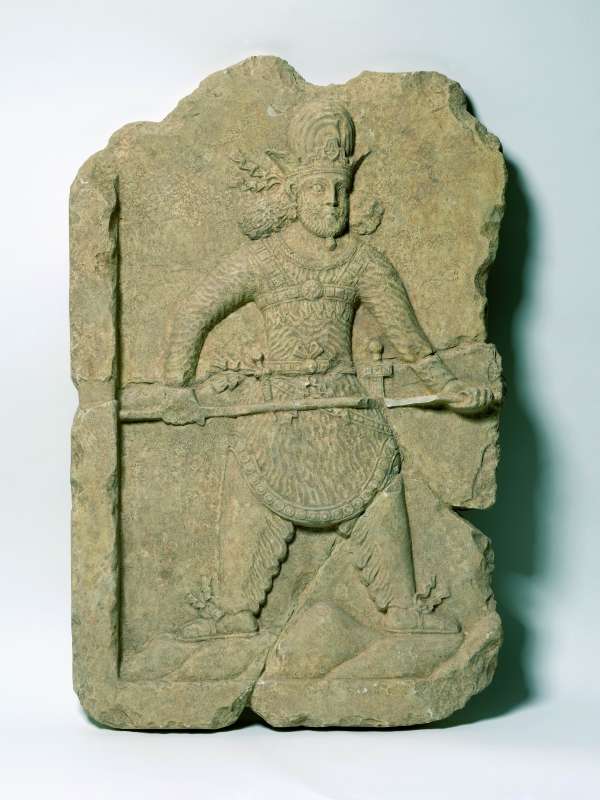The image depicts an ancient stone carving that stands upright against a completely white background, with a shadow cast to the right. The rectangular stone slab features a jagged top and a slightly uneven right edge. The central figure in the carving is that of an old-fashioned warrior, possibly from the Babylonian era or a similar time period. The warrior is depicted with a long, poofy beard and hair, wearing a distinctive dome-shaped helmet adorned with a crown-like embellishment. He is dressed in a loose, overall-type garment with frayed pants and cloth shoes tied with large cloth strips. The warrior holds a spear in his right hand while the tip of the spear is grasped in his left hand, as if drawing it from a sheath. The carving shows intricate details such as blade protection and the ornate nature of his helmet and attire. The warrior appears to be looking towards the right with a fierce expression, evoking a sense of historical grandeur and ancient craftsmanship.